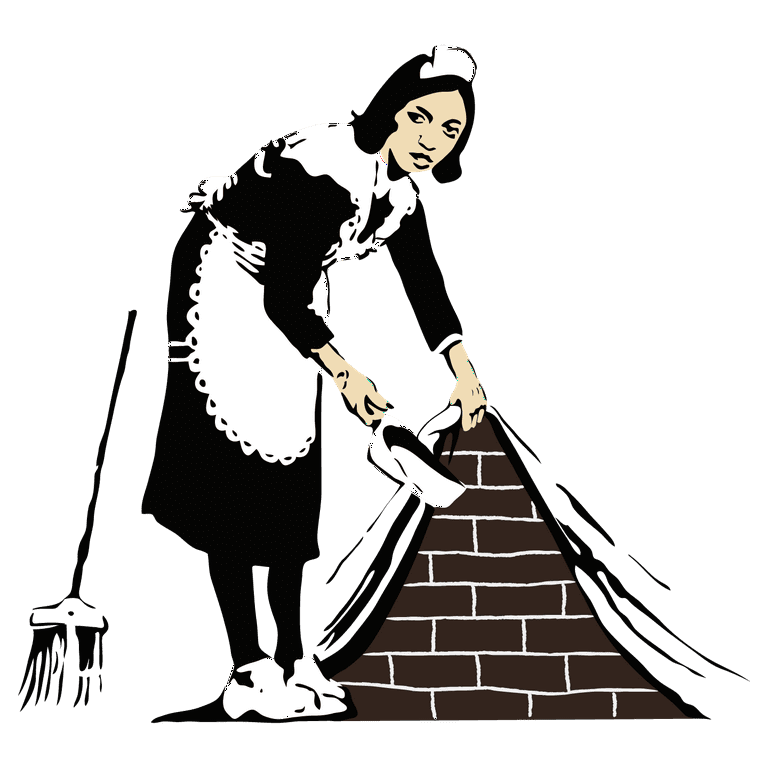The illustration depicts a maid in a classic French maid’s outfit, complete with a frilly apron, a little white hat, and a long-sleeved black dress. The majority of the image is rendered in black and white, with the only color being the pale yellowish tint of the maid’s skin and the brownish bricks of the brick wall. The maid, with a short bob haircut, is depicted holding a dustpan in one hand and lifting a portion of the wall with the other, revealing it to actually be a curtain that unveils the bricked surface underneath. To her left is a broom. The scene suggests she is about to sweep or dispose of the collected dust behind the curtain, giving an impression of revealing something hidden or mysterious. The stark white background contrasts sharply with the detailed drawing, making the maid and her actions the clear focal point. The piece bears a remarkable resemblance to the style of Banksy, capturing the enigmatic and subversive essence often attributed to his works.